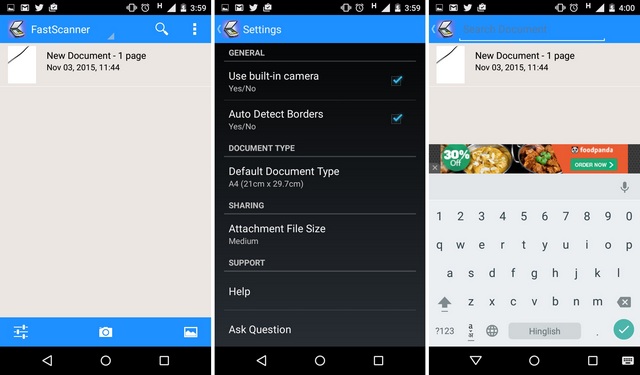The image consists of a collage of three separate smartphone screenshots displaying a tool named "Fast Scanner." 

The first screenshot features a user interface with a blue bar at the top labeled "Fast Scanner." Below it, a section titled "New Document, One Page" is visible, accompanied by a timestamp marked as November 3rd, 2015, 11:44. Adjacent to this text is a white rectangle. At the bottom of the screen, a blue rectangle houses icons for adjustments, camera, and photos. Beneath this are the standard navigation icons: a back arrow, a circle, and a square.

The second screenshot is labeled "Settings" at the top in blue. The background is predominantly black, adorned with white text detailing various settings options: General, Use Built-in Camera, Auto Detect Borders, Document Type, with Default Document Type set to A4, Sharing, Attachment File Size set to Medium, and Support sections including Help and Ask Question.

The third screenshot mirrors the first with its blue title bar reading "New Document, One Page" and the same timestamp. Midway down the screen, there is a visible advertisement for food. Below the ad, a pop-up keyboard is present, providing options for text, numeric, and emoji inputs. The bottom of this screen also features the standard navigation icons: triangle, circle, and square within a black rectangle.